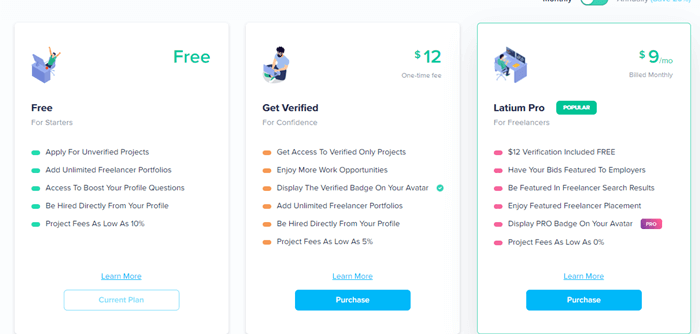The image captures a detailed price comparison chart set against a very light blue background. The chart is divided into three columns, each enclosed in white rectangles with different pricing plans.

The first pricing plan, positioned on the left side, is marked as "Free for Starters." The top right corner of this section highlights in green text the word "Free." The features, listed in black text with green bullet points, include:
- Apply for unified projects
- Unlimited freelancer portfolios
- Access to boost your profile questions
- Be hired directly from your profile
- Project fees as low as 10%

The second pricing plan is described in the middle column. In the upper right-hand corner, green text indicates a "$12" one-time fee. The left side, in black text with orange bullet points, lists the features:
- Get verified for confidence
- Get access to ratify-only projects
- Enjoy more work opportunities
- Display the ratify badge on your avatar
- Add unlimited freelancer portfolios
- Be hired directly from your profile
- Project fees as low as $5

The third and final pricing plan is on the right, titled "Lady M Pro, Popular." It features a green rectangular label. In the top right corner, green text states "$9 per month, billed monthly." The left side highlights the plan features in black text with pink bullet points:
- $12 ratification included free
- Project fees as low as 0%

The overall layout provides a clear, comparative view of what each plan offers.